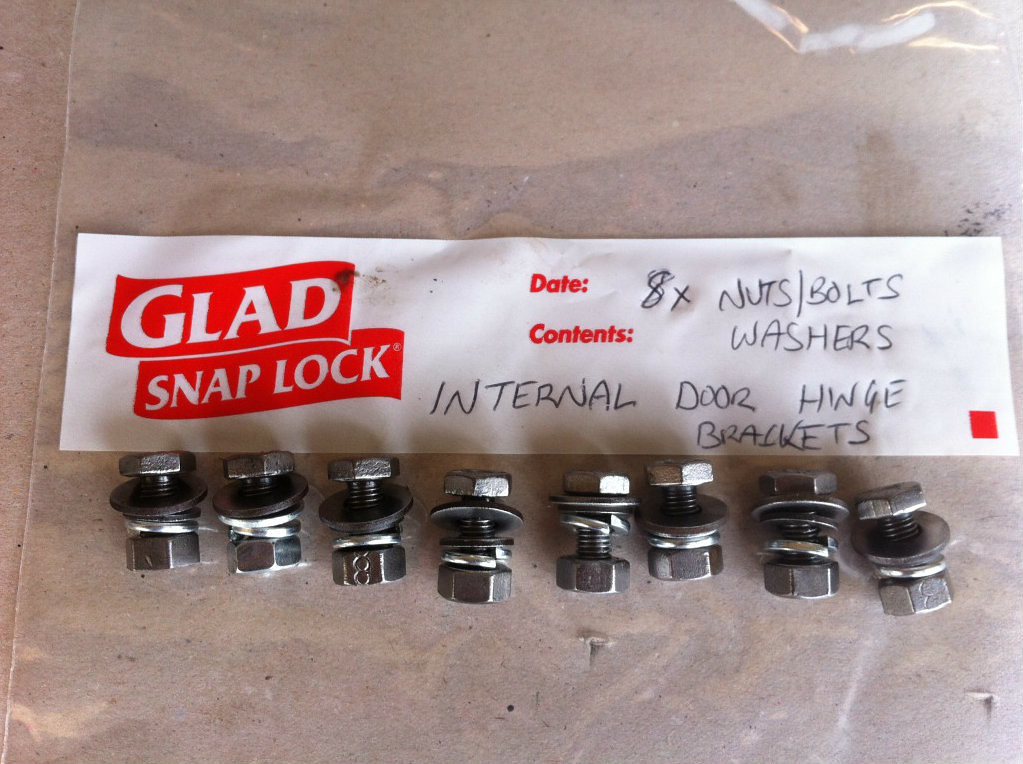The image depicts a photograph of internal door hardware components placed inside a GLAD Snaplock bag. The bag, which rests flat on a piece of card, contains eight individually assembled sets of nuts, bolts, and washers alongside internal door hinge brackets. The bag features a distinctive design with a red ribbon-like logo bearing the white text "GLAD SNAPLOCK." To the right, there's space labeled "DATE" and "CONTENTS," with the latter section hand-labeled in black pen as "8x NUTS/BOLTS WASHERS" and "INTERNAL DOOR HINGE BRACKETS." A small red circle appears at the bottom right of the white label area. The hardware items are neatly organized within the bag, which is clearly intended to keep them grouped together and easily identifiable for future use.